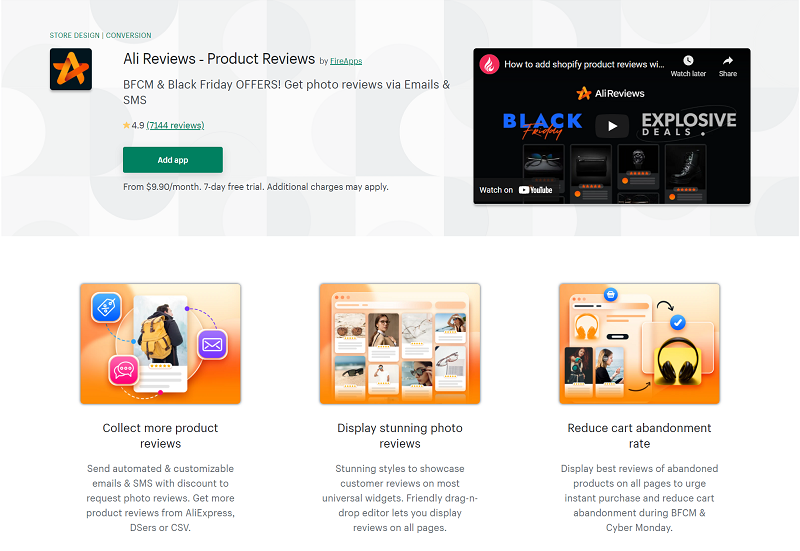This is a detailed description of a website homepage for "Ali Reviews - Product Reviews," featuring an option for users to download an app. The top left corner displays the categories "Store, Design, and Conversion," with an A and a star intertwined beneath it on a black background. The website promotes Ali Reviews, highlighting its features for BFCM and Black Friday offers, and the ability to get photo reviews via email and SMS. The service boasts a 4.9-star rating based on 7,144 reviews and offers a green "Add App" button, priced at $9.90 per month with a 7-day free trial and potential additional charges. To the right, there is a screenshot of the Ali Reviews interface, showcasing a Black Friday ad with explosive deals in a black and grey theme. This is part of an embedded video, complete with a play button, watch later, share options, and a link to watch on YouTube. Below, three columns with screenshots highlight key features: "Collect more product reviews," "Display stunning photo reviews," and "Reduce cart abandonment rate," each followed by a descriptive paragraph. Users are encouraged to click through to improve their e-commerce conversion rates.